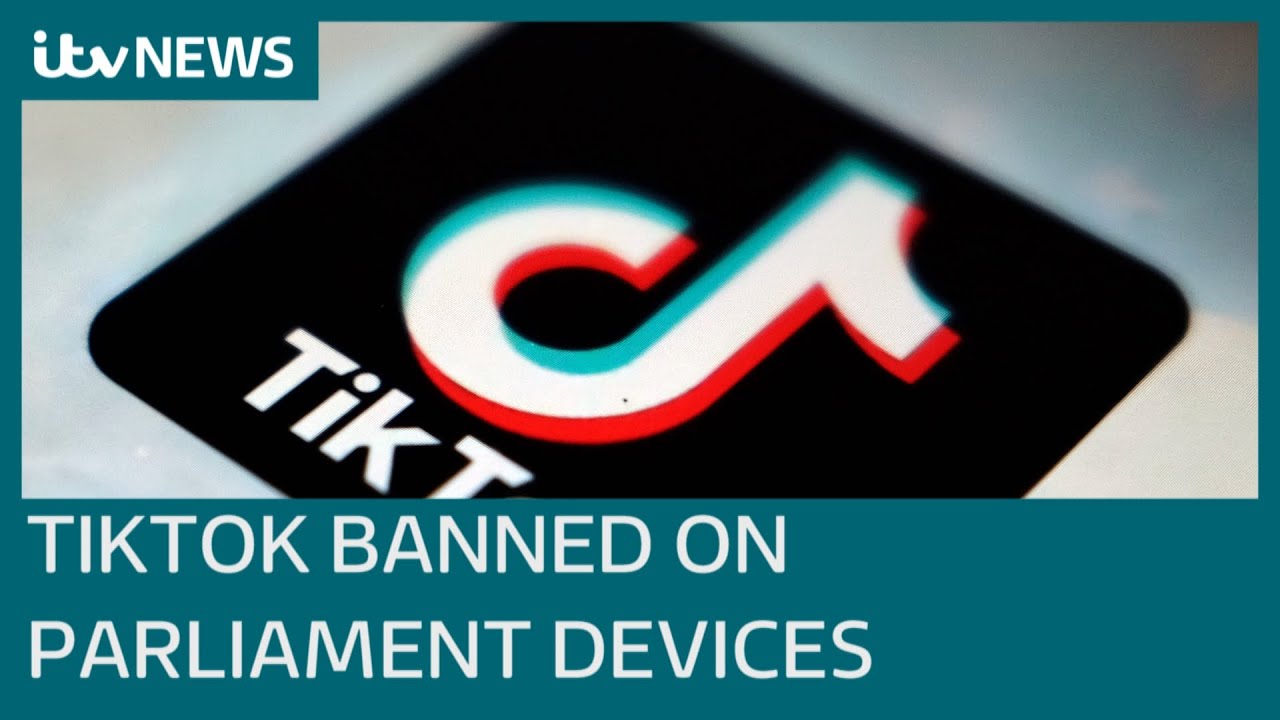The image is a horizontally-oriented teal rectangle with a teal frame. In the upper left corner, there is a small teal rectangle with white text reading "ITV News." Dominating the top two-thirds of the image is a photograph of the TikTok logo, which features a black square background with the TikTok symbol in green, white, and red. The word "TikTok" is partially visible, with only the word "tick" and a portion of the "T" showing. Below this photograph is a teal band with white, all-caps text stating "TIKTOK BANNED ON PARLIAMENT DEVICES."

The background of the TikTok photograph is blurred and features muted gray, blue, and reddish hues, focusing attention on the clear and vibrant TikTok logo. The overall colors in the image include teal, white, green, red, black, gray, and muted shades of blue and red.